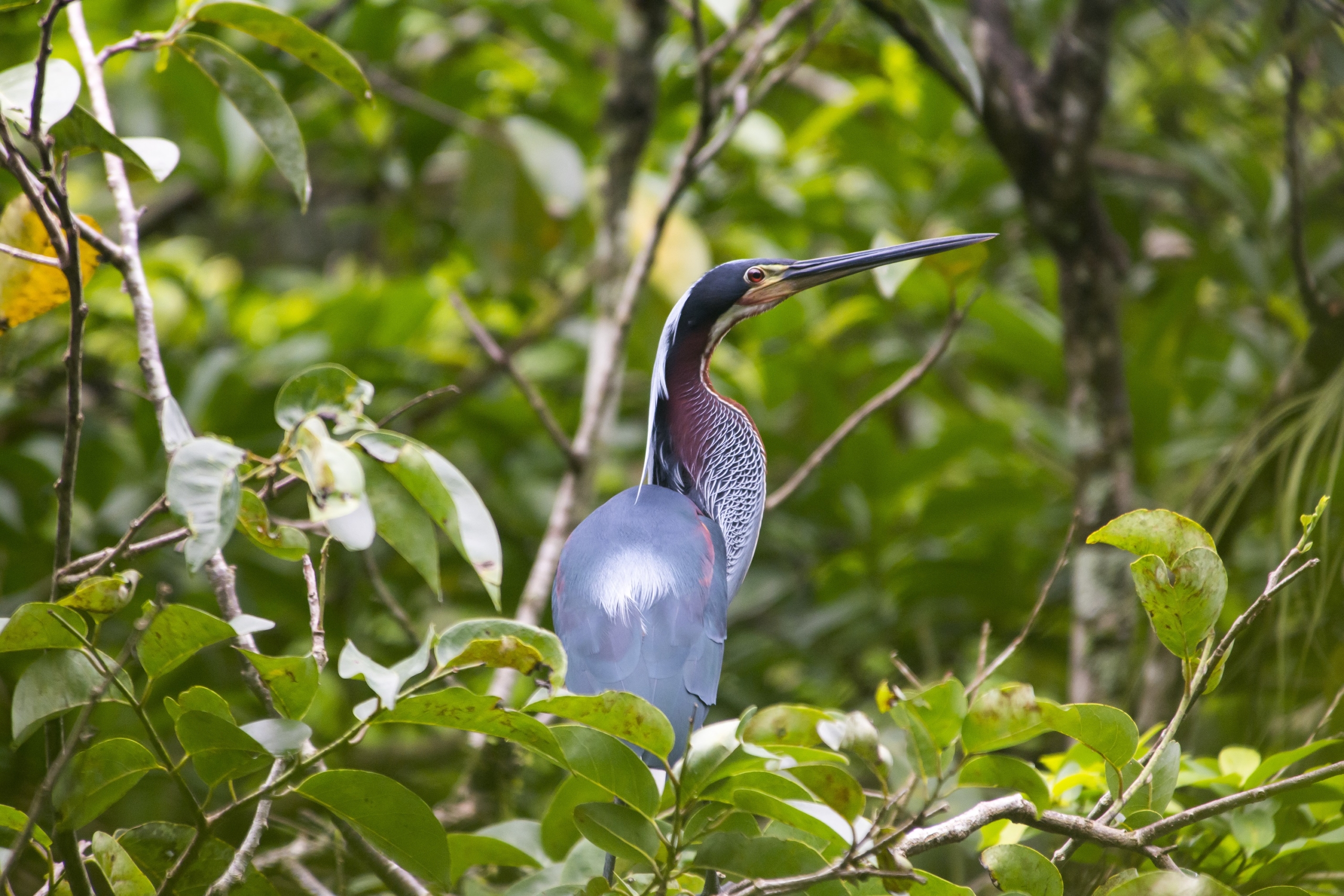A vivid photograph captures a bird perched in a dense thicket of greenery within a forest. The bird, which is facing away but has its head turned at a 45-degree angle to the right, displays a striking, elongated beak. Its shimmering silver body transitions to a darker gray with subtle hints of purple and blue around its neck and head. One eye, a reddish-brown color, peers towards the camera. The bird’s large, curved wing is an impressive blue-gray with a splash of white at the center, adding to its intricate coloration. The background is a blur of green leaves, plants, and narrow tree trunks, emphasizing the natural forest setting. The image radiates an outdoor, daytime atmosphere, capturing the bird stationary amidst the lush environment.